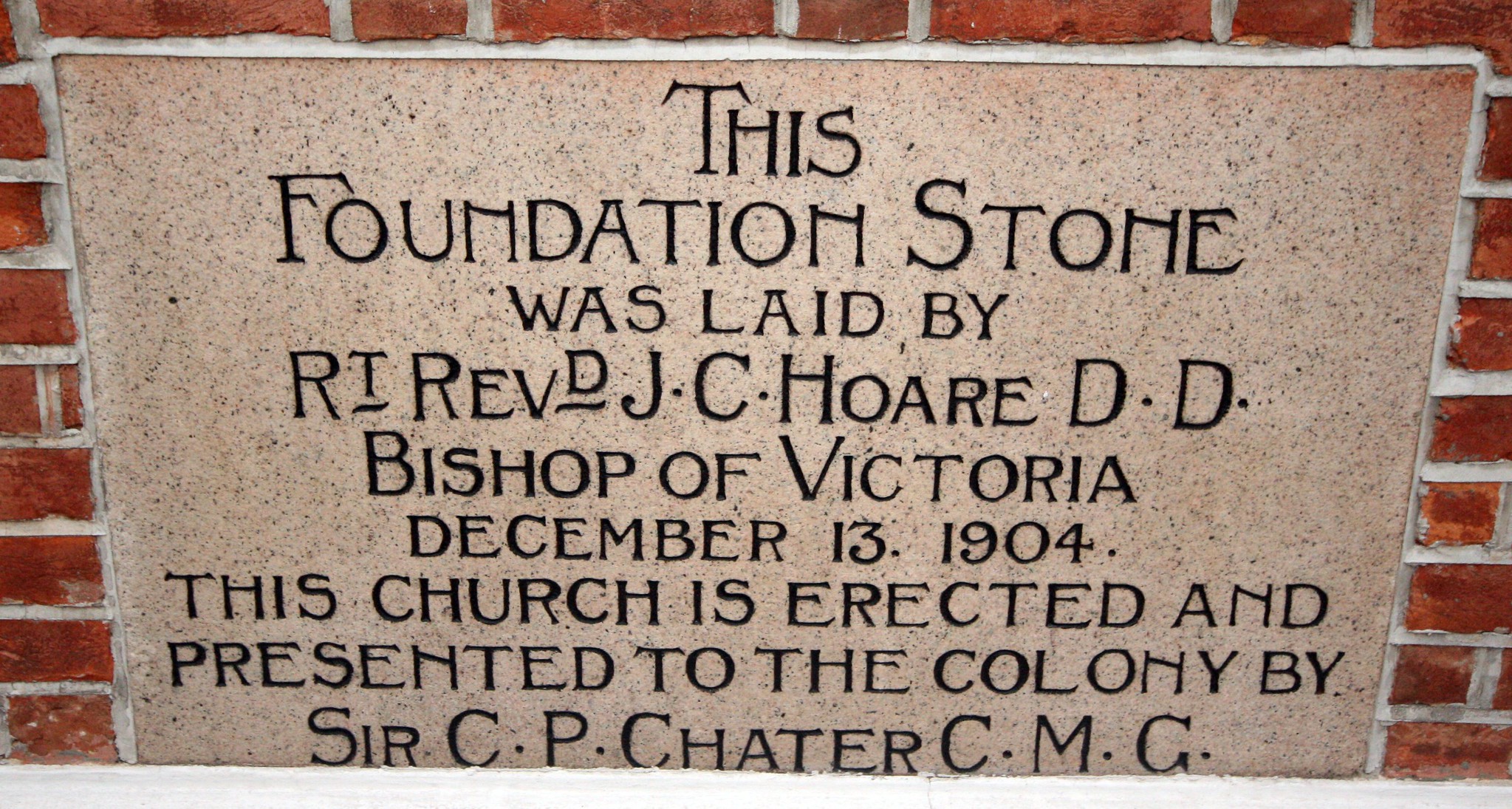The photograph, taken outdoors, depicts a historic foundation stone set into a red brick wall with a prominent brick-like design. The foundation stone is light red or pink in color and has a smooth, possibly marble or brownstone surface. The inscribed text, in all caps and black Century Gothic font, details the following: "This foundation stone was laid by Retired Reverend D.J.C. Hoard, D.D., Bishop of Victoria, December 13, 1904. This church is erected and presented to the colony by Sir C.P. Chatter, C.M.G." Notably, the letter 'T' in "Retired" and the letter 'D' in "Reverend" have lines underneath them, which adds a distinct detail to the stone.